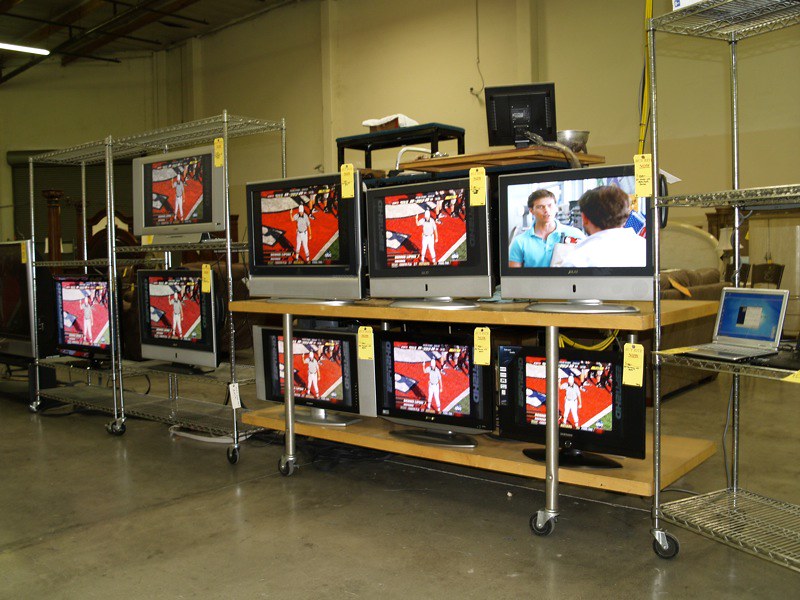A detailed photograph captures a dimly lit warehouse setting, showcasing four mobile carts laden with flat-screen TVs. Three of the carts are constructed from steel with wire grates, while the second cart from the right stands out with its orangey wooden shelves. The mannequins of consumer electronics, the TVs range in size from approximately 24 to 30 inches in diameter, with the majority featuring black and silver borders that suggest an older design, some completely black. Yellow price tags are affixed to the top right corners of each TV, hinting they might be for sale.

Starting from the left, the first steel cart supports two TVs. Adjacent to it, on the wooden cart, six TVs are neatly arranged with three on the top shelf and three below. The third cart, also steel, holds two TVs, one on each of its shelves. The rightmost steel cart is home to a solitary laptop on the top shelf and two plain black TVs on the bottom shelf. In the backdrop of this industrial tableau, a brown couch sits behind the wooden cart, and the warehouse's vast interior is hinted at by the visible beams and support structures on the ceiling. The floor is smooth, shiny concrete, and the plain beige walls contribute to the stark, utilitarian ambiance.